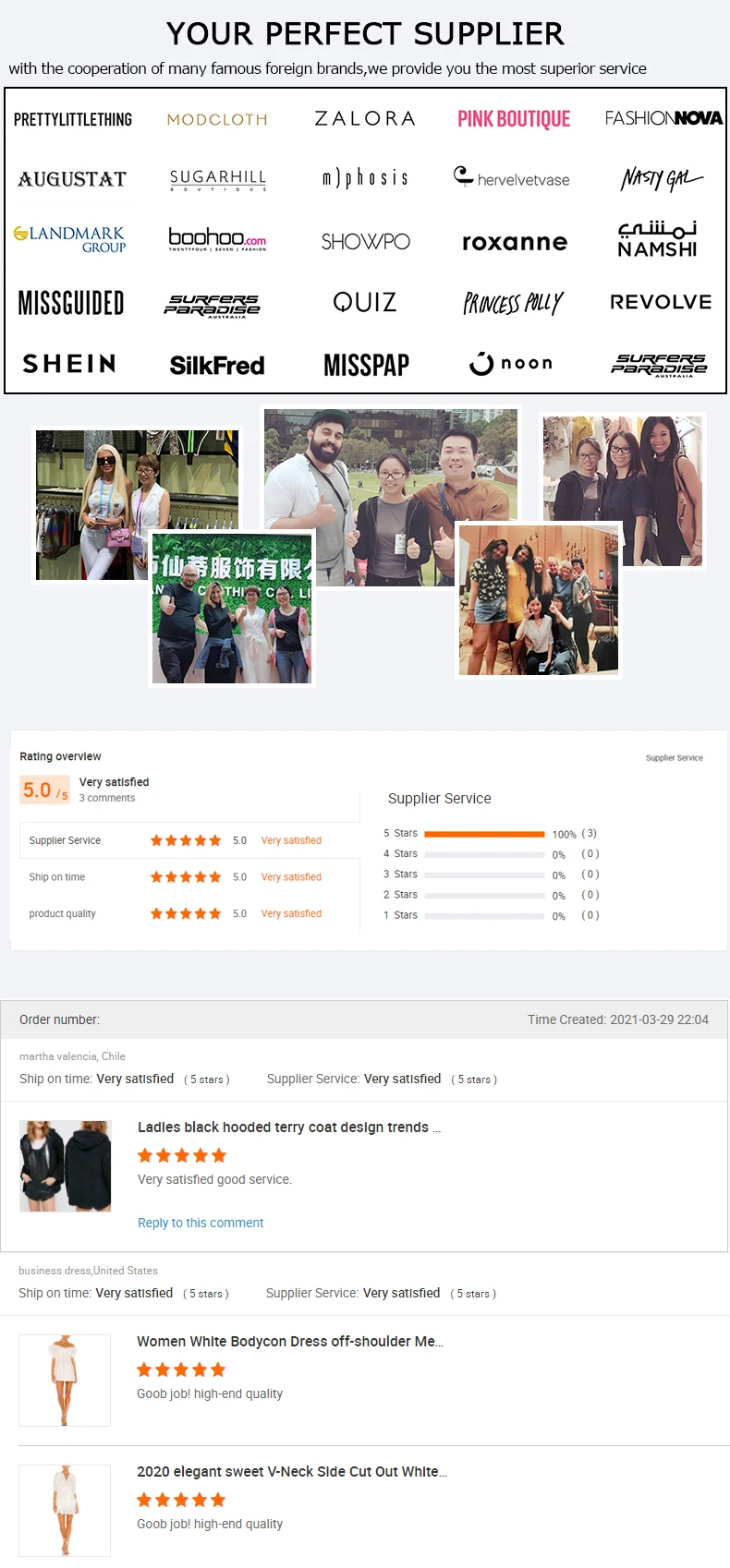Top Part: 

The top section of the site features a gray background with a black center. In the middle, a bold statement in all capital letters reads, "YOU'RE A PERFECT SUPPLIER." Beneath this headline, in standard black text, it states, "With the cooperation of many famous foreign brands, we provide you the most superior service."

Middle Section (Brands): 

A prominent white rectangular box with a black outline showcases various brand logos arranged in columns from top to bottom, left to right: 
1. Pretty Little Thing, Augustette, Landmark Group, Missguided, Shein
2. ModCloth, Sugarhill, Boohoo, Silk Thread, Service Paradise
3. Zalora, Morpheus, Showpo, Quiz, Miss Pap
4. Pink Boutique, Hair Velvet Vase, Voxan, Princess Polly, Noon
5. Fashion Nova, Nasty Gal, She, Revolve, Surface Paradise

Bottom Part (Reviews): 

Below the brand logos, five pictures of smiling individuals, mostly of Asian descent, are displayed, giving a personal touch to customer satisfaction.

Further down, there's another white rectangle that says "Rate and Review." Here are the featured reviews:

1. "Very satisfied, five out of five." - Reviewer 1
2. "Very satisfied" - Reviewer 2
3. "The woman's white bodycon dress off shoulder. Good job, high-end quality." - Reviewer 3
4. "2020 Elegant Sweet V-neck side cut white. Good job, high-end quality." - Reviewer 4

This detailed layout not only highlights the diverse range of collaborated brands but also showcases customer satisfaction through authentic reviews and relatable imagery.